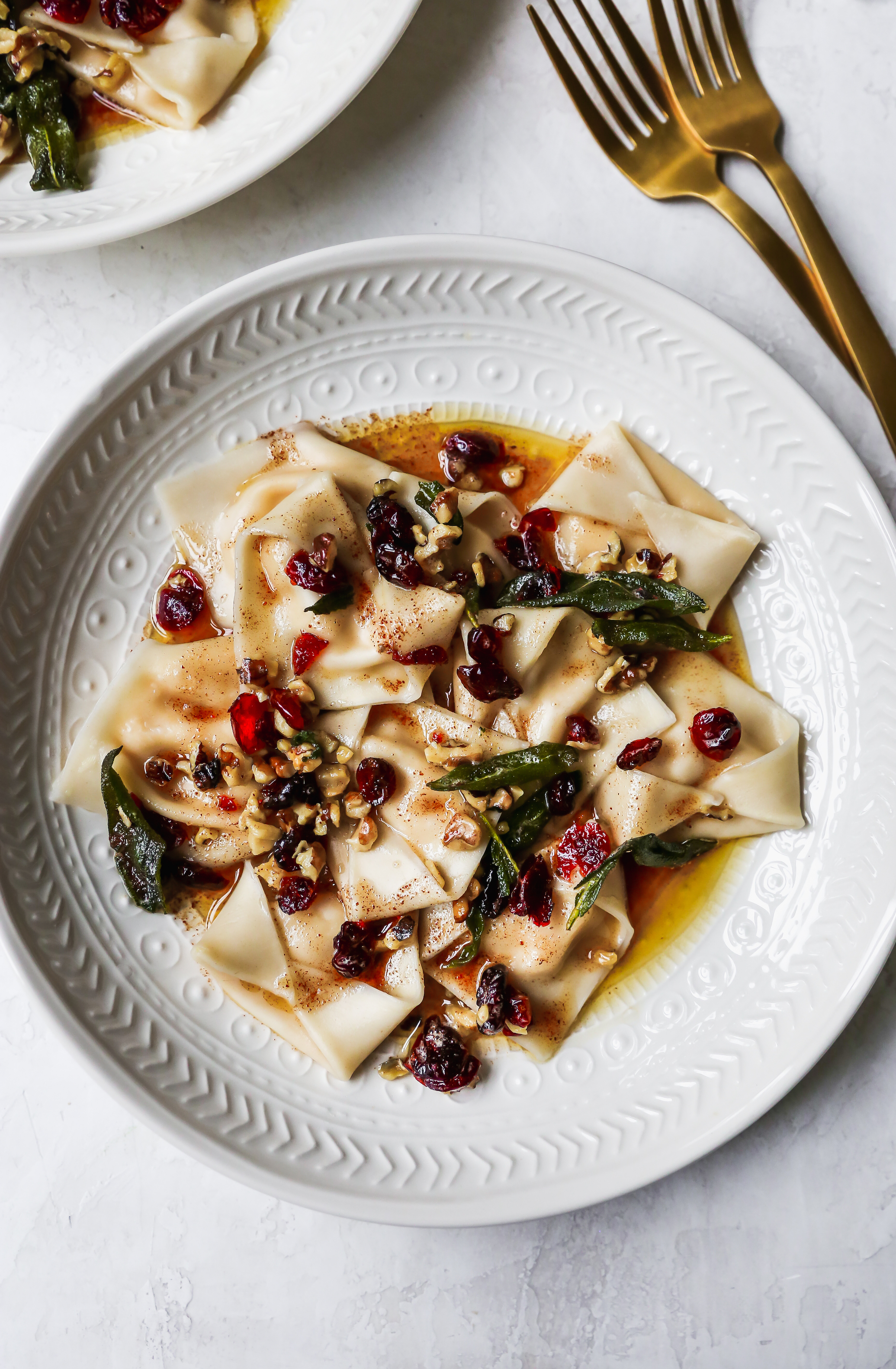The photograph reveals a meticulously arranged table setting featuring a richly detailed dish. The tablecloth and the china are both white, with the plates showcasing an intricate embossed edging composed of arrows, circles, dots, and a dashed line. At the center, the main plate holds a serving of wide, irregularly shaped noodles, bathed in a reddish-brown, oil-based sauce that appears to be a Sichuan or spicy chili oil concoction. Intermingled with the noodles are vibrant red berries or perhaps cranberries, along with green elements resembling anchovy or similar herbs. Additionally, the dish is garnished with crushed chili peppers, adding a spicy zest to the visual. There's a generous smearing of a red, jelly-like substance on the plate, enhancing the dish's vividness. To the upper right, two elegant gold forks lie beside the plate, and the edge of another plate with the same meal peeks from the top left corner. The composition is viewed from above, capturing both the artistry and the appetizing nature of the presentation.